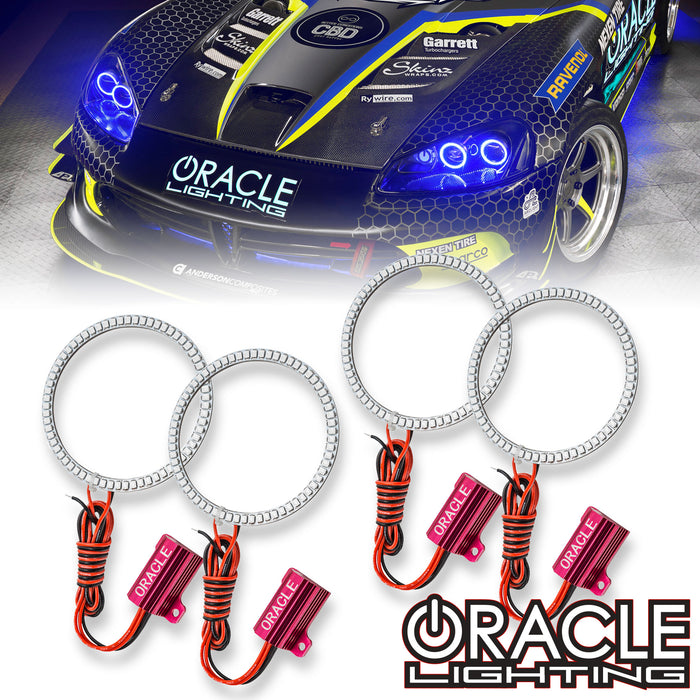This image is a detailed product photo in portrait orientation, combining photographic realism with graphic design elements. It features the front end of a sleek, black car reminiscent of a NASCAR vehicle, emblazoned with various sponsorship logos. Prominently displayed on the hood is "Oracle Lighting" in white text. The car showcases a black and silver honeycomb vinyl wrap extending across the hood, bumper, and front fenders, intersected by blue and yellow stripes running from the sides to the center-front. Yellow accents are also present around the fender. The headlights feature distinctive white rings emitting a bluish light, augmented by two blue LED circles in each headlight. The lower section of the photo fades into an arrangement of four LED rings, akin to those in the headlights, each connected via black and red cords to small pink controller boxes labeled "Oracle." The Oracle Lighting logo appears again in the bottom right-hand corner in white letters outlined in black. The car appears to be parked indoors, as suggested by the flooring beneath it.